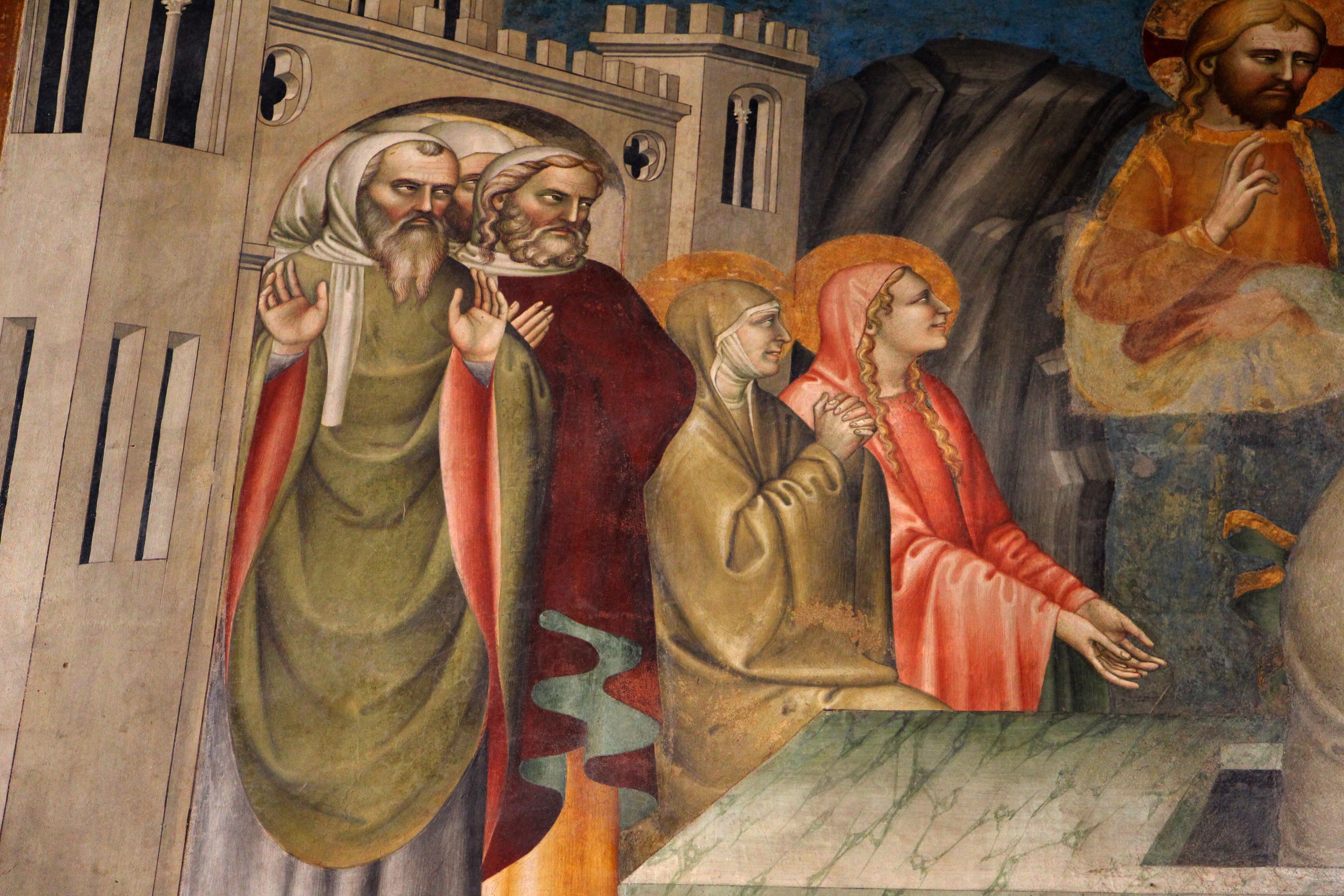The painting titled "Resurrection of Lazarus" by Giovanni da Milano and Matteo di Piccino, circa 1363-66, depicts a deeply religious scene evoking the Renaissance era. In the upper right-hand corner, Jesus, dressed in a brown shirt with long, curly hair, floats above, gazing off to the side. Below him stand two women, central to the composition: one in a prayerful pose wearing a greenish nun's habit, and the other, to her right, clad in a pink cloak with long blonde hair, also looking up at the floating Jesus. They are positioned in front of what appears to be a marble countertop. On the left side, three men in hooded cloaks with white headdresses emerge from a white building, their expressions a mixture of curiosity and agitation, directed toward Jesus. The background is a blend of blues and grays, complementing the white castle-like structure with dark mountains visible in the distance. The scene is imbued with a sense of solemn reverence, underscored by the varied emotional expressions on the figures' faces, ranging from wary to serene.